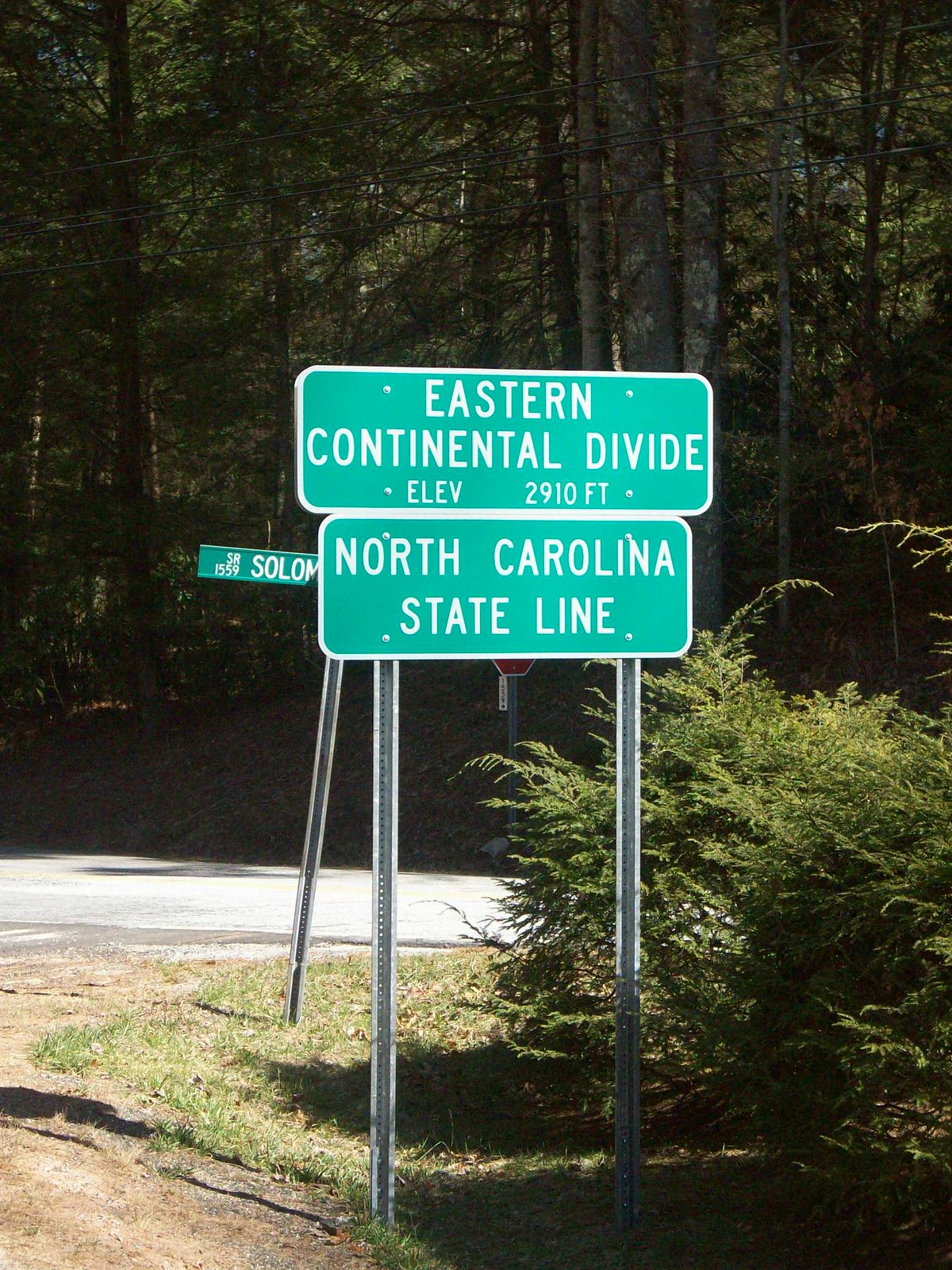The image depicts a set of road signs mounted on a single corrugated metal strip with punched holes for rigidity. The primary signs are green with white lettering; the top one reads "Eastern Continental Divide, Elevation 2,910 feet," while the one beneath it states "North Carolina State Line." To the right of these signs, there is a "Stop" sign and another smaller sign that seems to indicate "Solomon Street, SR 1559." The scene includes a mix of natural elements, such as grass, ferns, and tall pine trees just beyond the small road that diverges into a gravel or dirt path. The area appears quiet, possibly a rural or less-trafficked section, with a wooded background providing a serene backdrop to the road signs. Sparse greenery and a large bush mark the corner where these signs stand, emphasizing the tranquil setting.